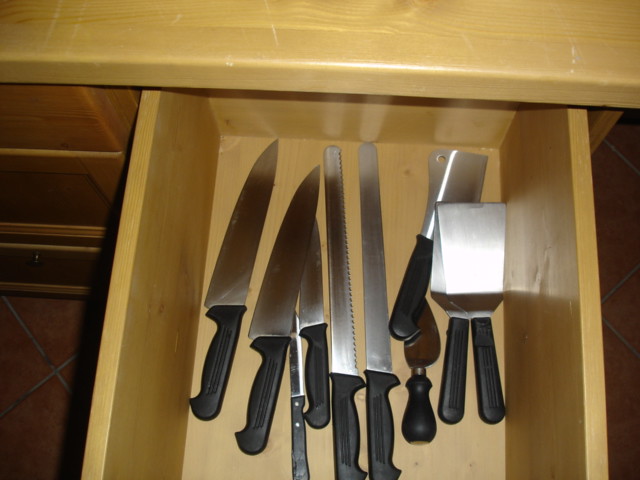This image is a detailed photograph of an open kitchen drawer, captured in a home kitchen setting. The drawer, centrally positioned in the frame, is pulled open to reveal an assortment of kitchen utensils. It contains approximately ten tools, including two large butcher knives, a small steak knife, another thicker but short knife, two long thin knives, and a meat cleaver, all characterized by their black handles and silver metal blades. Additionally, there is a mallet, a small spreader, and two spatulas positioned on the far right. The utensils are neatly arranged with blades facing upward toward the top of the image.

The drawer itself, as well as the surrounding cabinetry, appears to be made of a light, plasticky wood laminate, mimicking real wood but with a smooth, artificial finish. The countertop above the drawer matches this light wood laminate and also looks quite polished and synthetic, contributing to an overall uniform and modern aesthetic. The surrounding environment includes additional closed drawers in a darker wood tone, featuring soft edges that complement the kitchen's design.

The photograph is taken from a top-down perspective, and the flash was used, creating noticeable glare on the metallic surfaces and casting shadows, enhancing the detailing of the utensils. Elements of the kitchen floor are visible in the corners of the image, showcasing red tile arranged in a diamond pattern. The overall scene suggests an organized and well-kept kitchen space, with the primary focus on the neatly arranged drawer contents.